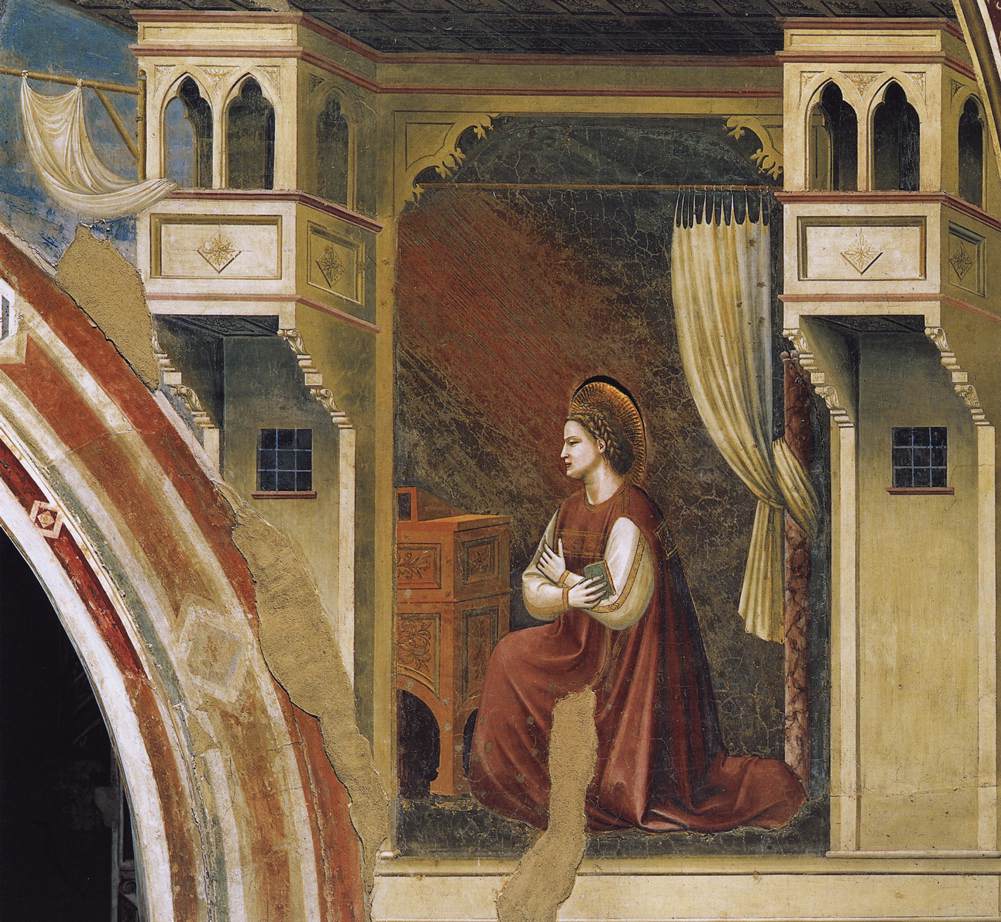In the center of this richly detailed painting, a regal figure, likely male, is seated on what appears to be a stage set mock-up of a castle. The focal point of the painting, this figure is dressed in an ornate maroon gown with golden sleeves and wearing a grand headdress adorned with intricate decor, extending several inches above the head. The hands are crossed at the chest, with the right hand holding a small book, which is green in color. The figure gazes stoically to the left side of the image.

The setting around the figure suggests an opulent, royal room with great design and architecture. The backdrop includes a dark green and red wall with patterned details, small windows, and a royal-looking cabinet with intricate designs. A pole with a rolled-up curtain is visible behind the figure, adding to the room's elaborate decor. Additionally, the painting seems aged, with visible signs of damage, including torn areas. The overall color palette includes black, white, red, gold, tan, orange, yellow, and blue, adding to the painting's antique and theatrical feel.